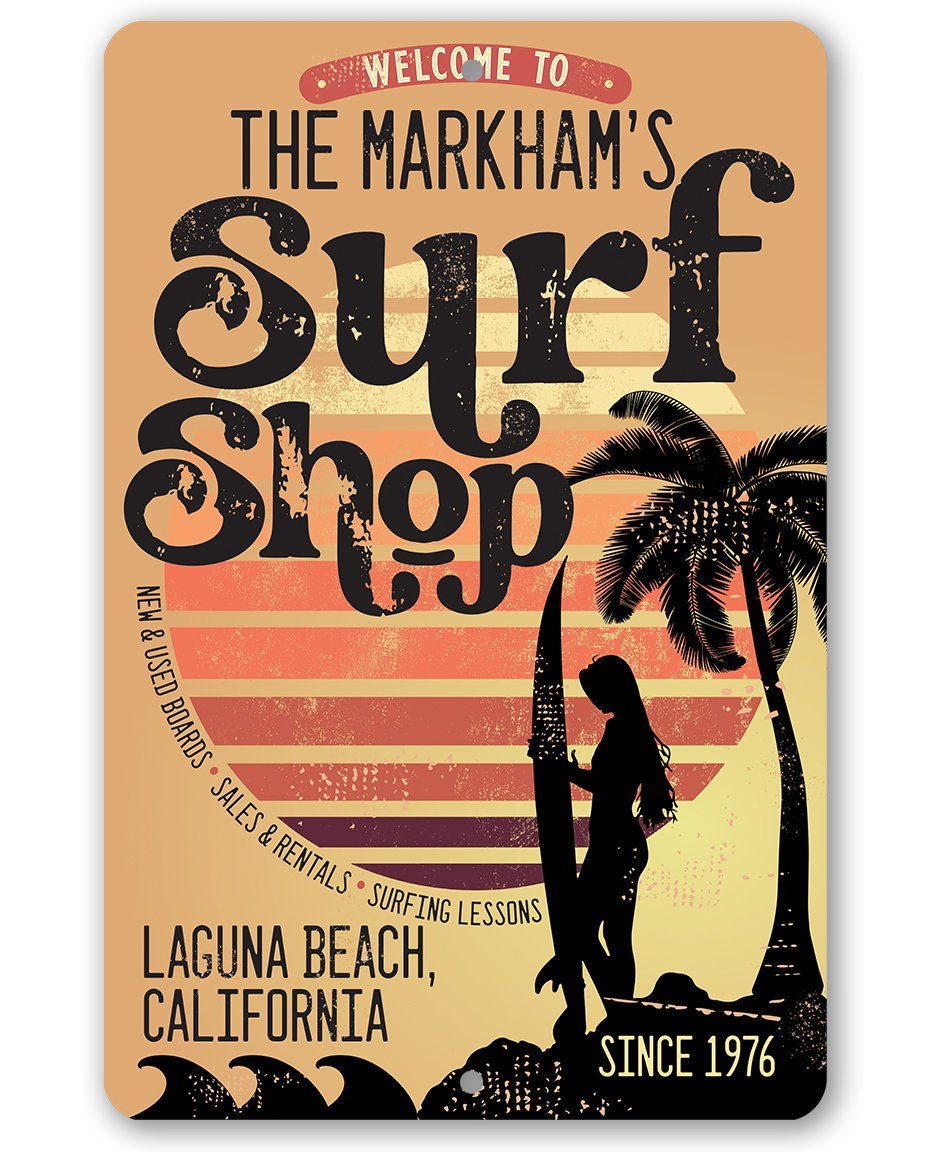This image depicts an advertisement for Markham's Surf Shop in Laguna Beach, California, designed to resemble a classic, worn ticket or sign with a vibrant and nostalgic aesthetic. The rectangular card has rounded corners and a hole at the top, indicating it could be attached to a lanyard. The background features a gradient transitioning from yellow at the top through orange to a darker red at the bottom, with the top half of the card adorned by a large, artistically rendered sun. The sun is depicted with horizontal stripes that shift from yellow at the top to a deeper red at the bottom.

At the top of the card, a red banner with the text "Welcome to" in white introduces the shop. Below that, in fancy black lettering designed to look roughly printed, it reads "Markham's Surf Shop." Around the sun, black text announces "New and Used Boards, Sales and Rentals, Surfing Lessons." This is framed by a silhouette of a female surfer holding a surfboard vertically, standing on a small island under a palm tree with small cartoony ocean waves at the very bottom. This silhouetted scene is located in the bottom and right quadrants of the card, adding to the tropical and beachy vibe.

Additional text at the bottom left corner reads "Laguna Beach, California," while the bottom right corner indicates the establishment year "Since 1976." The intricate mix of colors, retro design, and thematic elements make this a striking and detailed visual representation of the surf shop.